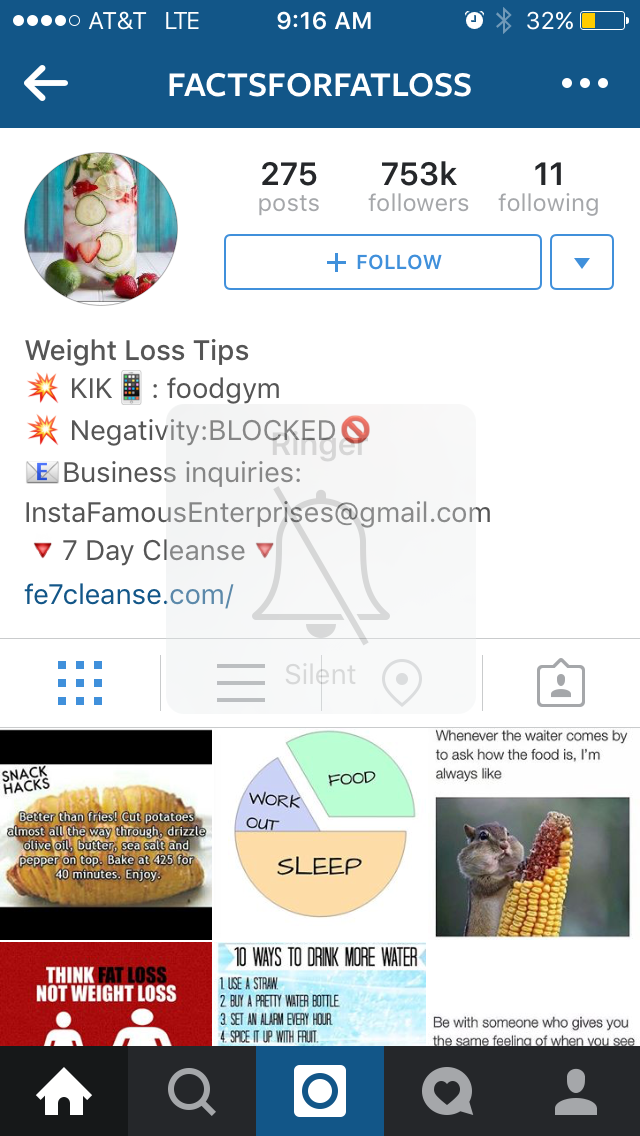This image is a tall, rectangular screenshot from a cell phone, displaying an Instagram account page under the service provider AT&T at 9:16 AM with 32% battery remaining. At the top, a dark blue bar features an arrow pointing left, reading in white capital letters "FACTS FOR FAT LOSS" next to three vertical dots. Below this, on a white background, the Instagram profile features a circular image of a cup filled with various fruits, followed by a white and blue "Follow" button and another button pointing downwards. The account has 275 posts, 753K followers, and 11 following. The profile description includes "weight loss tips," "kick: Food Gym," "negativity blocked," "business inquiries: instafamousenterprises@gmail.com," and a link to "7daycleansefe7cleanse.com." Below the bio, six thumbnail images are displayed for scrollable content, including sections on snacks hacks, a split diagram of workout (top left), food, and sleep (largest portion), and tips for drinking more water. The screen's bottom row features icons: a house, magnifying glass, round button with a heart inside, and a profile silhouette.